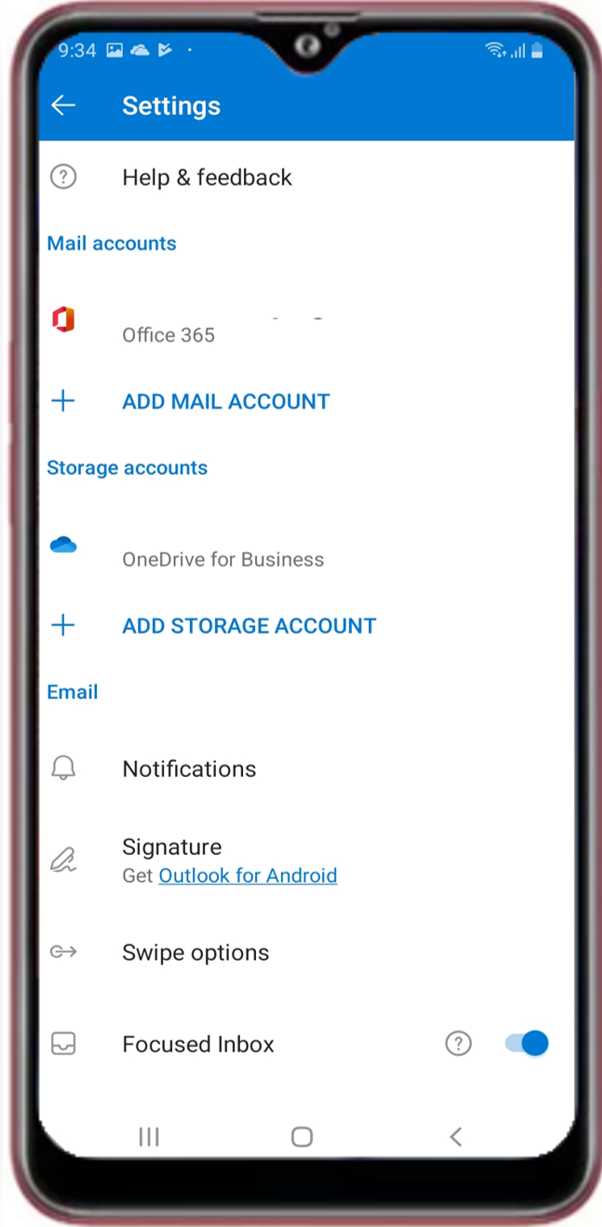The image displays a cell phone with its Settings page open. At the top of the screen is a blue banner with the number "934" prominently displayed. The banner also contains three icons: a photo icon, a cloud icon, and a triangle with a checkmark inside it. In the top-right corner, icons indicating Wi-Fi connectivity, mobile data, and a battery icon showing half charge are visible.

Centered on the banner, a white back arrow and the word "Settings" are clearly displayed. Below this, against a white background, various options are listed:
- Help and Feedback
- Mail Accounts
- Office 365
- An option to add a mail account indicated by a plus sign
- Storage Accounts
- OneDrive for Business with a plus sign to add a storage account
- Email Settings
- Notifications
- Signature settings
- An option to "Get Outlook for Android"
- Swipe Options
- Focused Inbox with a toggle switch highlighted in blue

At the bottom of the screen, three navigation icons are present: three vertical dots for options, a home button, and a back arrow.

The phone itself is enveloped in a black border with a silver spot at the top center for the camera. Surrounding this is a slight silver border followed by a thin red border encompassing the entire outer edge of the phone.